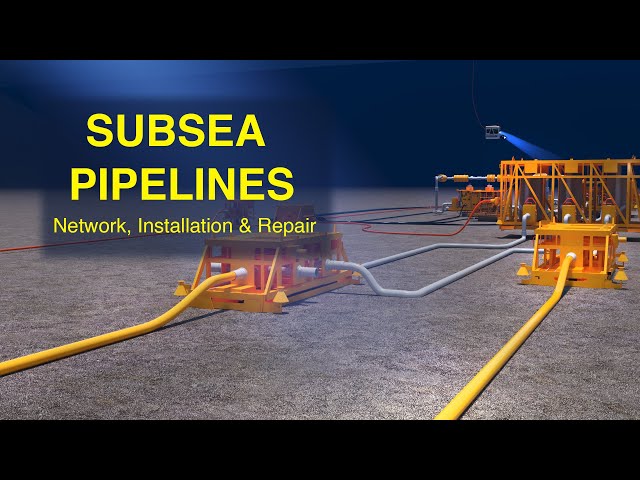The image is a detailed 3D artist's rendering titled "Subsea Pipelines Network Installation and Repair." Set against a backdrop of murky, deep blue ocean waters, the illustration shows a flat seabed, depicted in beige, where a complex network of pipelines is laid out. Various pipelines in colors like yellow, white, red, and blue are visible, with the yellow and white ones being more prominent. These pipelines connect to large, safety-orange-yellow, cage-like junction boxes. In the background, a deep sea diving vessel equipped with a light shines down onto the undersea installation, illuminating the scene, especially the yellow structures. This digital, animated sketch effectively demonstrates the configuration and intended functions of the subsea pipelines network, showcasing an advanced setup for installation and repair operations on the ocean floor.